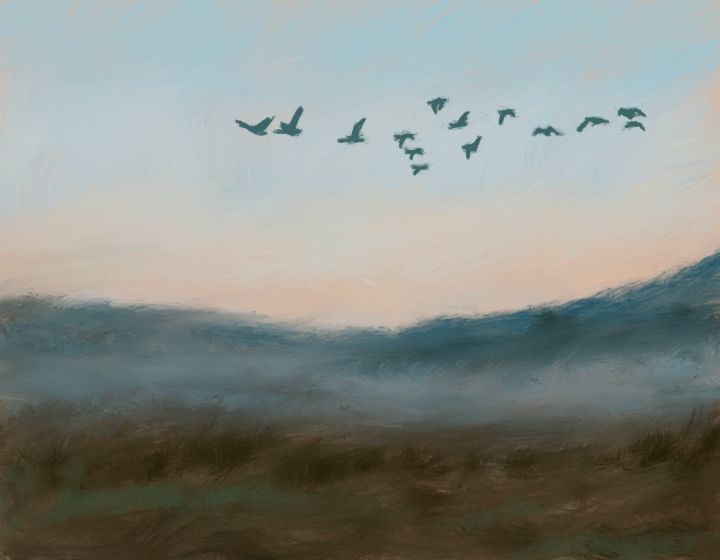The painting is a detailed, rectangular watercolor landscape with a ratio of 2:1 in width to height, executed on canvas or paper. The scene is impressionistic, featuring a textured, spiraling brown foreground suggesting earthy elements, transitioning towards a teal-tinted bottom. Rising from this, the landscape slopes gently upward with grayish-blue tones, before descending softly and merging with a colorful, evocative sky.

The sky mirrors the tranquility of dusk, starting with a light blue hue that gradates into a peachy orange near the horizon. The upper part of the sky is more prominently blue, with a flock of about 13 to 14 birds sketched in delicate gray or blue outlines, creating a dynamic focal point. These birds are clustered mainly towards the right and middle sections of the painting, soaring gracefully across the sky, their forms suggested more than detailed.

The painting's overall effect is a blend of soft color transitions and textured impressions that evoke the serene beauty of a landscape at dusk, with the birds adding a sense of liveliness and movement.